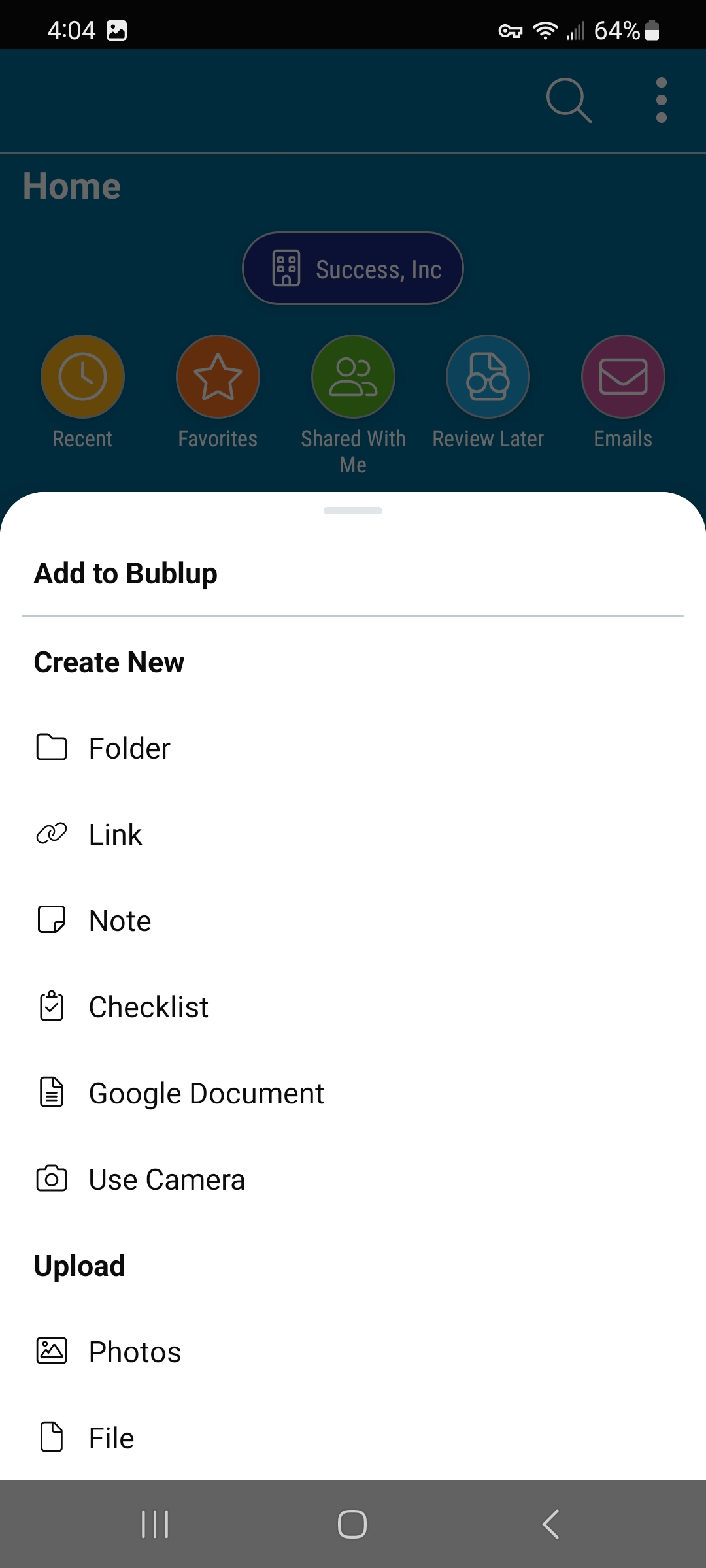In the image, we are looking at a screenshot set against a black background. In the upper left corner, the time is displayed in white, "4:04," along with an icon for photos. In the upper right corner, the Wi-Fi symbol is visible, indicating Wi-Fi is on, and the battery icon shows 64% remaining. Below, in a grayed-out section, there is a magnifying glass icon followed by a narrow, horizontal gray line. Beneath that, "Home" is displayed in bold text. 

Immediately below, there is a button labeled "Success, Inc." featuring an icon resembling a small apartment building. Under this button are five circles with icons, representing different actions: "Recent," "Favorites," "Shared With Me," "Review Later," and "Emails."

At the bottom of the screenshot, a white page is prominently displayed. At the top of this page, "Add to Bubble Up" is written in bold black text. Below this, the options "Create New" are presented, followed by choices in regular text such as "Folder," "Link," "Note," "Checklist," "Google Document," and "Use Camera."